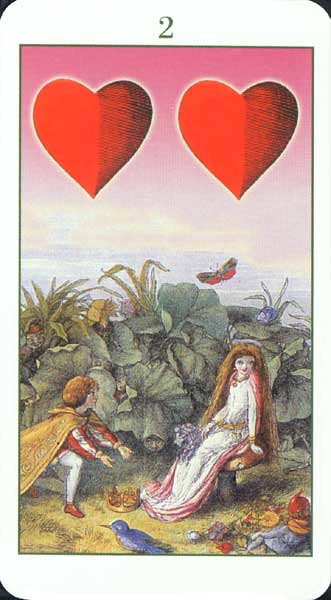The image depicts a tarot card with a detailed illustration. The card is tall and rectangular, slightly narrower than a standard playing card, with a white border and rounded corners featuring small black edges. At the top of the card, the number "2" is displayed in black. The central area of the card contains a tall rectangular illustration extending towards the bottom.

The illustration features a vibrant pink sky adorned with two large red hearts, each heart displaying a gradient with the left side bright red and the right side more shaded. Below the sky, lush green bushes and trees create a verdant backdrop. At the forefront of the scene, a woman sits gracefully on a mushroom. She wears a flowing white dress and a light brown veil, accessorized with gold bracelets and a gold belt. In her hand, she holds a bouquet of purple flowers.

Kneeling before the woman is a man, dressed in a red and white long-sleeve shirt and a yellow cape draped over his shoulders. He wears white tights, brown shoes, and has brown hair. With one knee on the ground, he extends his hands toward the woman. At her feet lies a crown, positioned just below the man's outstretched hands.

The bottom of the illustration showcases a grassy area where they stand. A blue bird perches in the center of this grassy expanse. In the right corner of the image, a collection of flowers and fruits, including apples, melons, and purple flowers, is artistically arranged in a piled display.